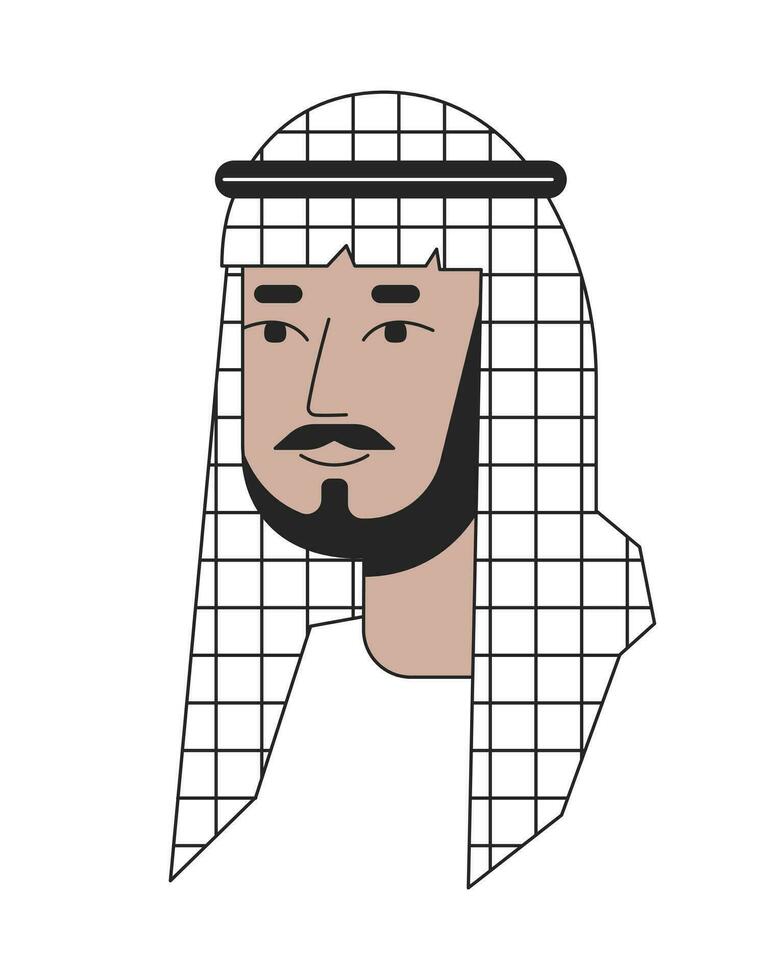The image portrays a Middle Eastern individual with a medium to deep brown, mocha-toned complexion. The person has a prominent black beard that frames their face, and their eyes are a striking dark brown. They are depicted with a flat, somewhat disengaged facial expression, adding a layer of intrigue to their appearance.